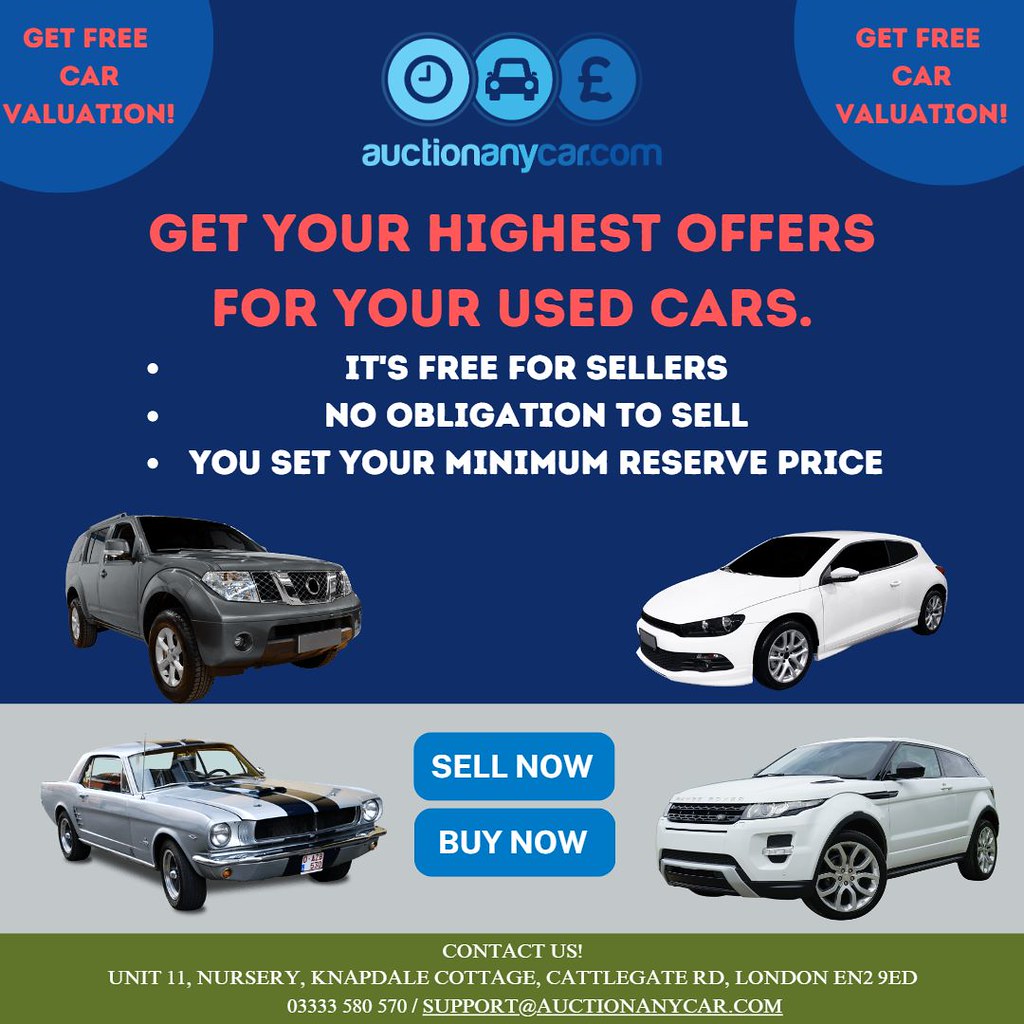This square advertisement predominantly features a dark blue background with various colorful text and elements aimed at promoting a car-selling service. At the center of the ad, in prominent orange text, it boldly states "Get your highest offers for your used cars". Underneath this headline, there are three bullet points in white text highlighting key features: "It's free for sellers," "No obligation to sell," and "You set your minimum reserve price."

The upper left and upper right corners of the ad feature red text within cut-off circles, both stating "Get free car valuation." Below the central content, images of four different cars are displayed: a Nissan Xterra, a Volkswagen Golf, a Ford Mustang, and a Range Rover. Amid these images, blue text buttons reading "Sell now, buy now" are strategically placed to catch the viewer's attention.

Towards the bottom, the ad has an olive green band that contains the company's contact information: "Contact us, Unit 11, Nursery, Napdale Cottage, Cattlegate Road, London, EN2 9ED," as well as a telephone number and email address. The website name, "auctionanycar.com," is displayed prominently at the top of the ad, tying all the elements together to inform potential customers about their car auction services.